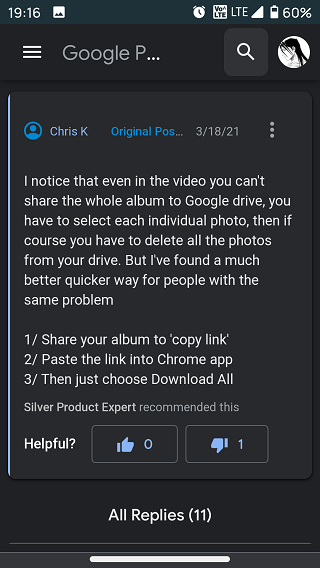This is a detailed description of a screenshot from a social media post viewed on a mobile phone with a dark theme:

---

The screenshot showcases a social media post on a mobile device, featuring a black background indicative of a dark theme. Across the top, a dark greenish-blue header bar displays various icons and information. The time is indicated as 19:16. Just to the right of the time, there is an icon containing a white square with two mountain peaks. On the upper right-hand corner of the header, several icons are visible: an alarm clock symbolizing a set alarm, a VoLTE icon within a white square, the text "LTE," a white triangle pointing right, and a vertically oriented battery showing approximately 60% charge, accompanied by the text "60%."

Below the header, a black bar contains three white horizontal lines, followed by the text "Google P..." suggesting a truncated title. To the right of this text is a white search magnifying glass icon nestled within a gray box with rounded corners. Additionally, there is a circle avatar characterized by a white background and the black and white image of a samurai or a man with long hair looking to his left.

The central content of the post, authored by a user named Chris K., is dated 3-18-21. The text, written in white and centered on the screen, reads:

"I noticed that even in the video you can't share the whole album to Google Drive. You have to select each individual photo. Then of course you have to delete all the photos from your drive, but I found a much better quicker way for people with the same problem. 1. Share your album to Copylink. 2. Paste the link into Chrome app. 3. Choose download all. Silver Product Expert recommends this."

At the bottom of the post, there is a prompt asking if the information was helpful, followed by two interactive buttons: a thumbs up button showing zero likes and a thumbs down button indicating one dislike. Additionally, text at the bottom indicates that there are "all replies (11)" available for viewing.